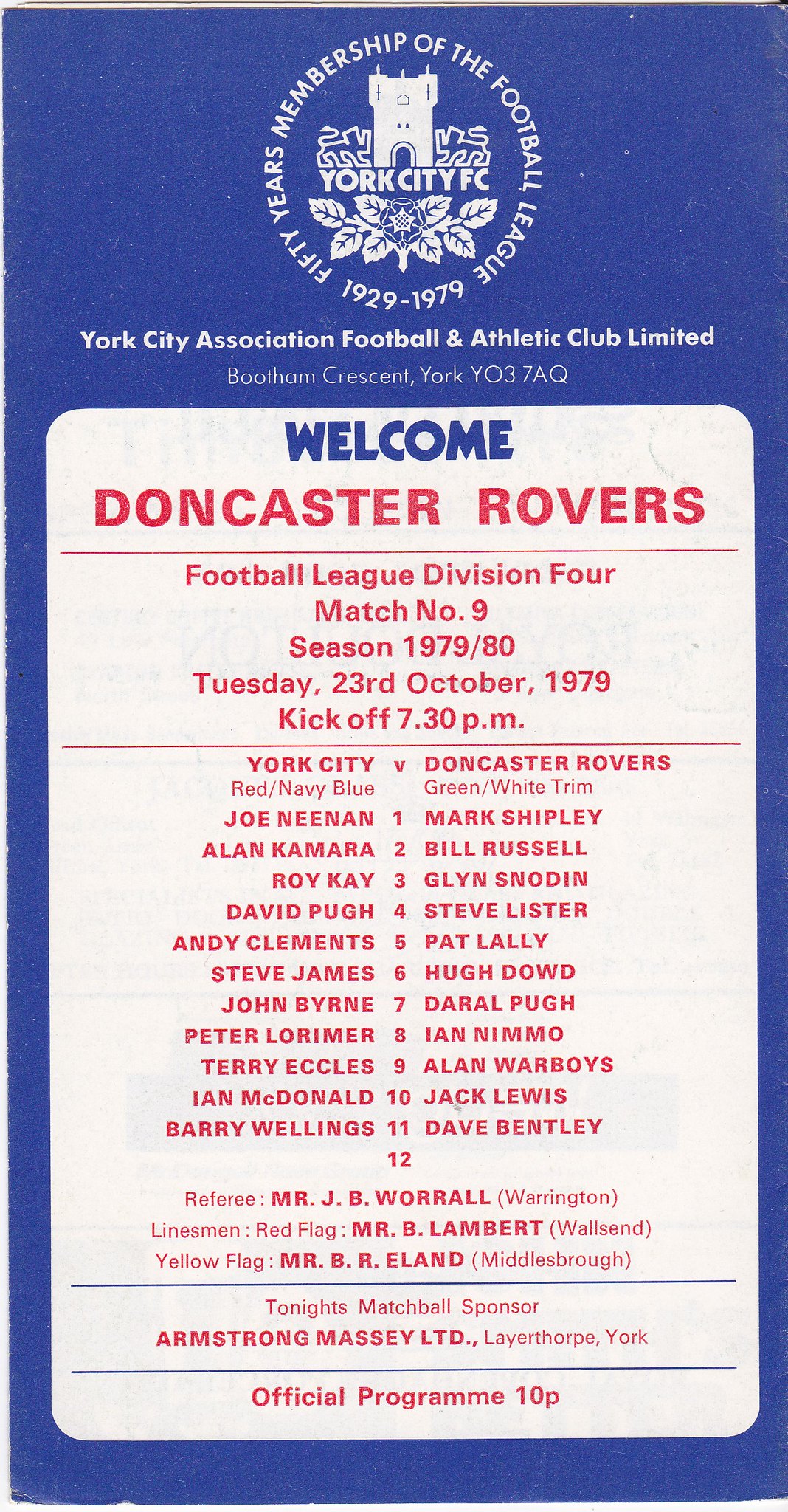The front page of an official soccer program features a dark blue background with a white middle section. At the top of the page, there's an emblem with the text "50 Years Membership of the Football League, 1929-1979." Below this, it reads "York City Association Football and Athletic Club Limited" with the address "Bootham Crescent, York, YO3 7AQ."

The central section welcomes the Doncaster Rovers for a Football League Division IV match, labeled as Match Number 9 of the 1979-80 season. The match is scheduled for Tuesday, 23rd October 1979, with a kickoff at 7:30 p.m. The text provides details on the team colors: York City in red and navy blue, and Doncaster Rovers in green and white trim.

Further down, the program lists the lineups for both York City and Doncaster Rovers, naming players such as Joe Neenan, Mark Shipley, Allen Camera, Bill Russell, Roy K., Glenn Snodden, David Pugh, Steve Lister, Andy Clements, Pat Lally, Steve James, and Hugh Dowd. Additional information includes the match referee, linesman, and the match sponsor, Armstrong-Massey LPB. This official program is priced at 10 pence.